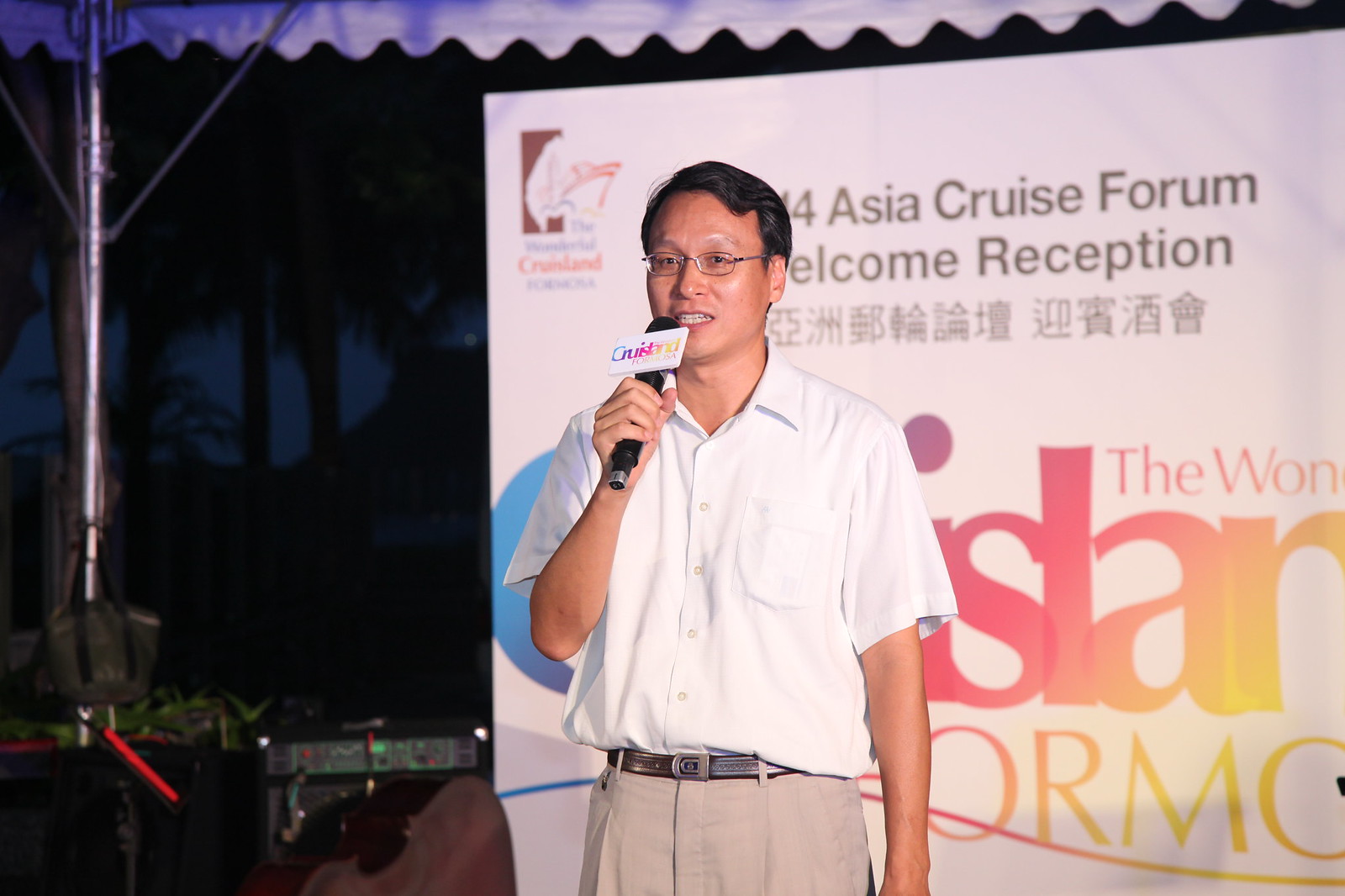In this detailed, full-color photograph, we see an Asian gentleman delivering a presentation at the Asia Cruise Forum Welcome Reception. The event takes place outdoor during nighttime under a white, wall-less canopy tent held up by silver metal poles. The man, standing at the center of the image, is dressed in khaki pants with a brown belt featuring a silver buckle, and a white button-up collar shirt with a chest pocket. He is holding a black microphone adorned with a logo or colored marking. Behind him, a white billboard serves as a backdrop, displaying the text "Asia Cruise Forum Welcome Reception" in bold black letters, followed by lines of Asian characters. Although some text near the end is obscured, the words "Island" or "Cruise" are partially visible. The scene is illuminated, highlighting the man's features and attire, while the dark skies and trees are faintly visible in the background.